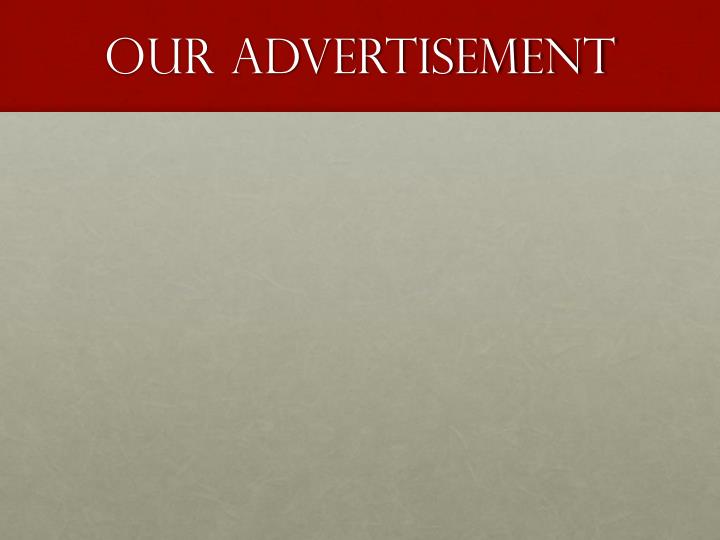The image depicts a minimalist advertisement slide designed for a computer slideshow. The top portion of the slide features a striking deep red rectangular strip that spans horizontally from left to right, covering roughly one-fourth of the total slide height. Centered within the red strip, in all-uppercase white letters, is the text "OUR ADVERTISEMENT," presented in a formal, narrow font that exudes a rich and expensive appearance. The bottom portion of the slide, occupying more than three-fourths of the space, is a solid medium gray color that is unembellished. This creates a stark contrast between the vibrant title strip and the muted background below, enhancing the minimalist aesthetic of the advertisement.